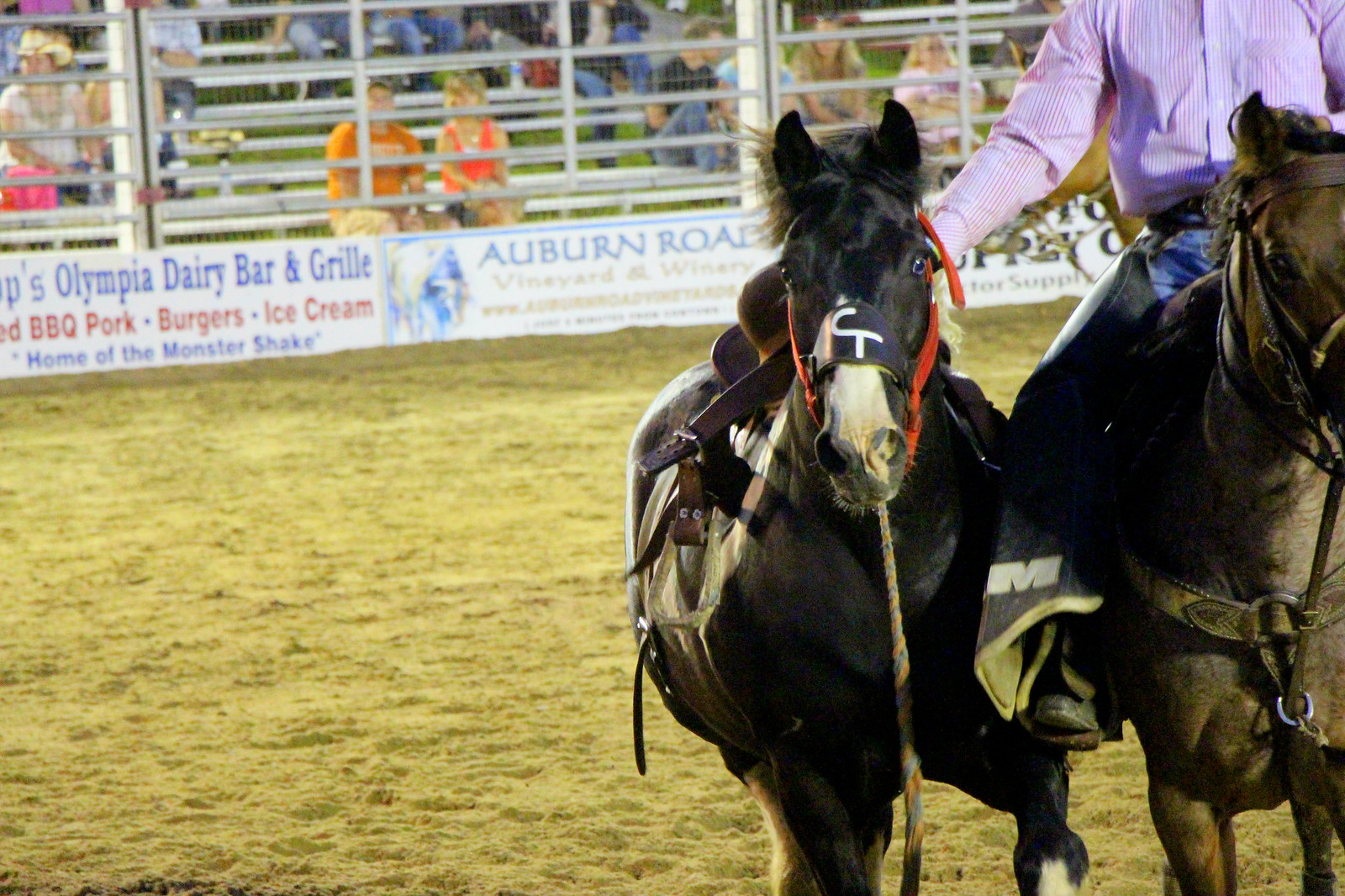In this photograph, we see two saddled horses in an arena, suggesting a rodeo or horseback riding show. The brown horse on the right is partially visible, being ridden by a man whose upper body is out of the frame. He’s dressed in blue jeans, chaps, boots, and a pastel-colored shirt, possibly pink, reflecting the bright sunlight. The rider extends his right hand towards the black horse beside him. The black horse, detailed with a white nose and a red bit, has striking blue eyes and is riderless. The arena's ground is brown dirt, bordered by metal poles and fences. Behind the fence, spectators fill the bleachers, attentive to the event. Prominent sponsor banners are visible, one reading "Olympia Dairy Bar and Grill" and another partially showing "Auburn Roads" amidst other words obscured by the scene. The image captures the vibrant atmosphere of the event and the beauty of the horses in a moment of action.